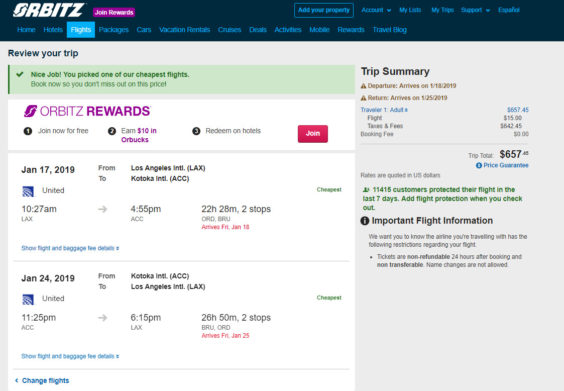The image depicts a webpage from the Orbitz website. The top navigation bar is predominantly black, featuring various options including Home, Hotels, Flights, Cars, Vacation, Partners, Careers, Activities, Rewards, and Travel Blog. The navigation options are blurry, making some of them hard to read clearly. 

The 'Flights' tab is highlighted, and a message encouraging the user to book their flight is prominently displayed: "Review your trip. Nice job! You picked one of our cheapest flights. Book now so you don't miss out on this price." 

Below this message is a promotional offer highlighted in purple, "Orbitz Rewards. Join now for free. Earn $10 in Orbitz, Redeem on Hotels," with a red button labeled "Join."

The details of the selected flight are partially visible, although some sections are obscured by blurriness. The flight is scheduled for January 17, 2019, from Los Angeles (LAX) to Kolkata International Airport (ACC). The airline is United, with a departure time of 10:27 a.m. from LAX and an arrival time of 4:55 p.m. at ACC. The total journey time is 22 hours and 28 minutes, with two layovers in Chicago and an additional city, which is unreadable due to the blur.